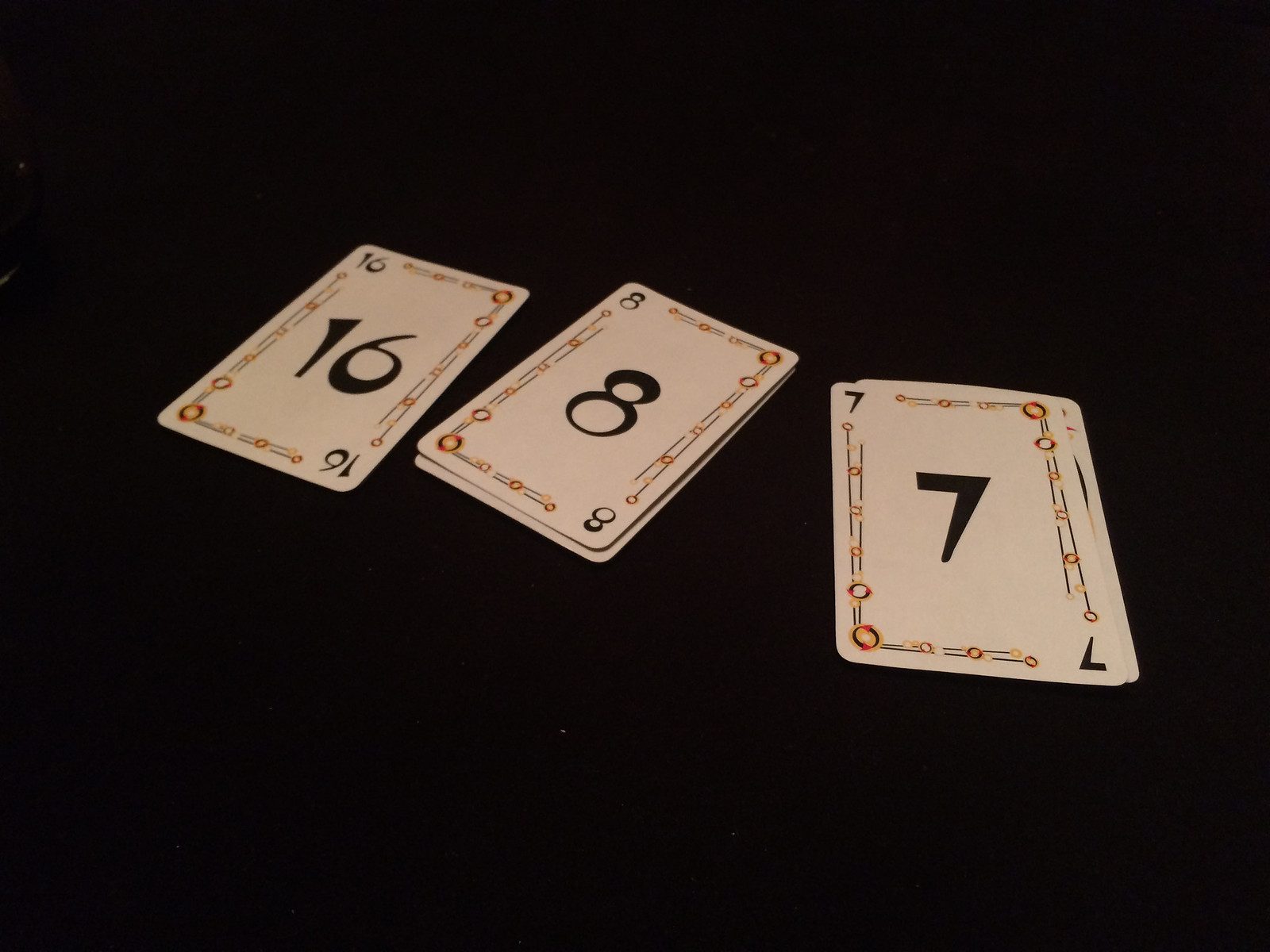The photograph showcases a central alignment of three playing cards, each marked by distinct number designations and a recurrent decorative theme. Positioned on the left is a card numbered 16, featuring an off-white background with a striking black "16" displayed prominently in the center, as well as in the top left and bottom right corners. The card is bordered by intricate patterns of gold circles intersected by black lines, giving it a rich, ornate appearance. 

At the center of the photograph is the number 8 card, also in off-white. The card's design mirrors that of the 16-card, with a bold black "8" at the center and repeated in the top left and bottom right corners, encased within the same decorative border of gold circles and black lines.

The card on the right is designated with the number 7, consistent with the design language observed in the previous cards. Its off-white canvas is marked by a black "7" located centrally, and again in the top left and bottom right corners. The same luxurious border of gold circles and black lines encapsulates the number.

The backdrop of the scene is a smooth, black surface, suggestive of a felt table often used in card games, adding a tactile context to the arrangement. The lower portion of the image hints at additional cards beneath, partially concealed by the trio above, maintaining the thematic border and numbering style observed in the visible cards.